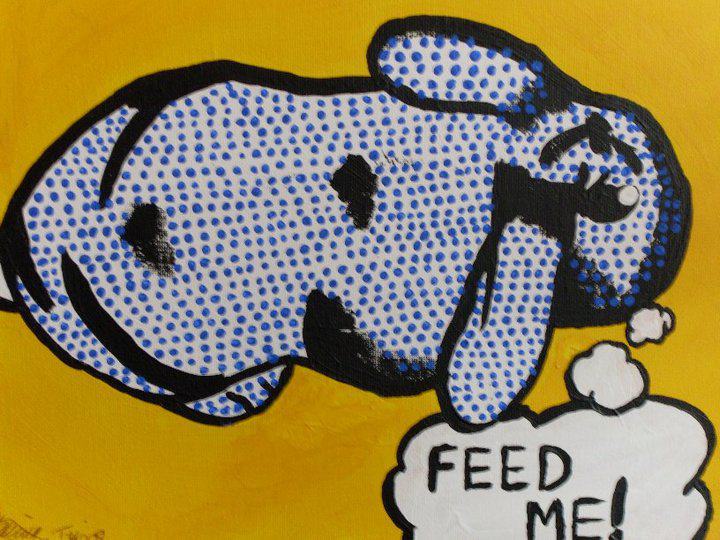This landscape-style image depicts a cartoonish rabbit rendered in a comic book-like illustration with heavy black outlines and a pointillist pattern of fine blue dots. The rabbit appears almost like graffiti, seen from a top-down perspective, and is placed against a vivid yellow background. The rabbit is captured facing right, with its right side more visible, and features floppy ears, beady black eyes, and little feet. Surrounding the figure are additional blue dots, maintaining the comic book aesthetic. A white thought bubble emerging from the rabbit contains the text "FEED ME" in black capital letters, adding to the whimsical nature of the illustration.